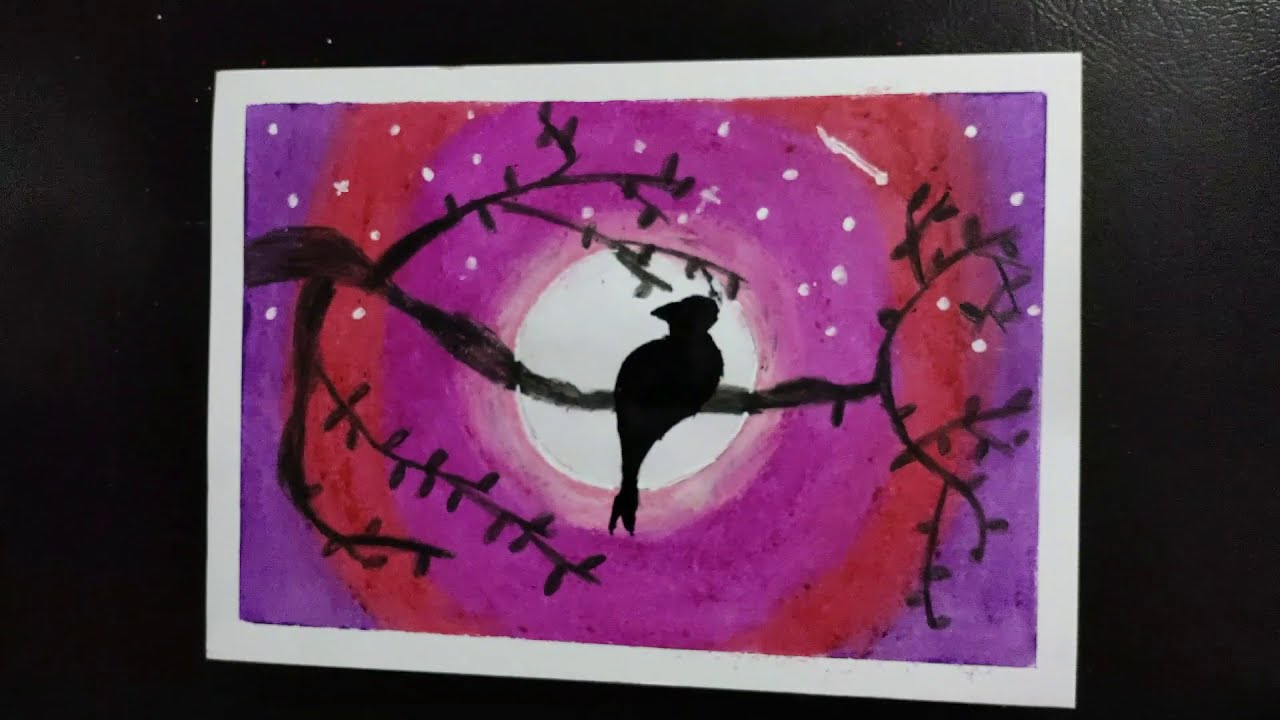The image features a black, textured background that resembles leather or pressed vinyl with a subtle groove and a shine from a light source on the right side. The main subject is a rectangular picture with a distinct white border. Inside the picture, a large, bright white moon occupies the center, surrounded by concentric rings of purple, pink, and light pink hues, with subtle reddish tones at the outermost ring. Scattered around the circular moon are small white stars, depicted as dots and X marks.

In the foreground, a black tree branch extends from the left side, adorned with sparse black leaves. Perched on this branch, directly in front of the moon, is the black silhouette of a creature. While it may be interpreted as a bird, its artistic rendering suggests it could also resemble a small dragon or a cat with a split tail, leaving some ambiguity about its exact nature. This image, likely a painting or print, captures an ethereal and mystical nocturnal scene with a strong use of contrasting colors and textures.